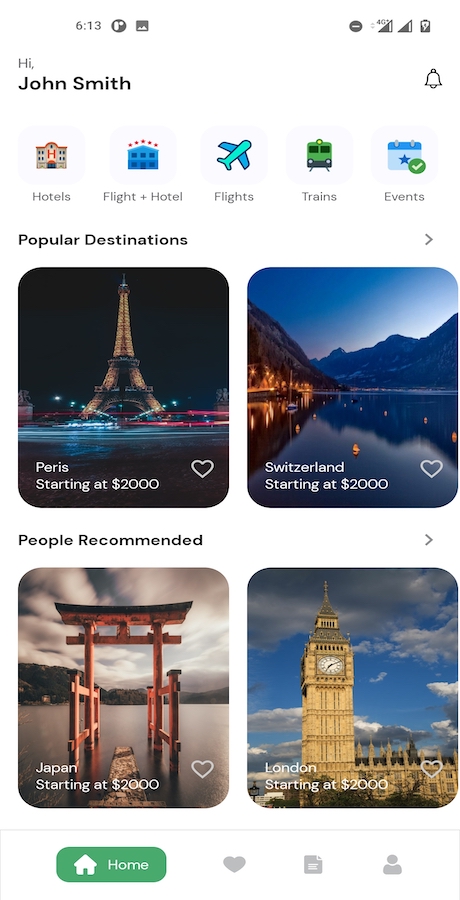A detailed and cleaned-up caption for the image could be:

"Displayed on the mobile phone screen is a travel app interface. At the top of the screen, the status bar shows the time as 6:13, alongside symbols indicating notifications and signal status. The phone has 4G connectivity and the battery is three-quarters full.

Beneath the status bar, a greeting message reads, 'Hi, John Smith.' Below this introduction, there are five colorful icons for different travel options:
1. A red 'H' icon indicating Hotels, possibly linked to hotels.com.
2. A blue building with five stars representing Flight + Hotel packages.
3. A blue airplane symbol for Flights.
4. A green train icon for Trains.
5. A calendar with a blue star and a green circle enclosing a white check mark labeled Events.

No specific option appears to be selected.

Further down, a header labeled 'Popular Destinations' is present, with a clickable arrow for more options. Featured destinations include:
- A stunning night view of the Eiffel Tower in Paris, labeled 'Paris' (misspelled as P-E-R-I-S) with trips starting at $2,000. A heart icon next to it allows users to like the destination.
- A picturesque scene of water, mountains, and lights labeled 'Switzerland' starting at $2,000, also with a heart icon.

Another section titled 'People Recommend' features additional destinations with clickable arrows for more options:
- An enchanting image of a pergola on the water in Japan, surrounded by mountains and cloudy skies, with trips starting at $2,000.
- A classic shot of Big Ben in London, starting at $2,000. Both have heart icons for users to like the trips.

At the bottom of the screen is a navigation bar. The 'Home' icon is highlighted in green with a white house symbol and text. Three grayed-out icons follow: a heart, a document with lines and a bent corner, and a person icon, potentially representing other sections of the app not currently active."

This caption is both comprehensive and descriptive, detailing all visual elements and potential functionalities depicted in the image on the phone.